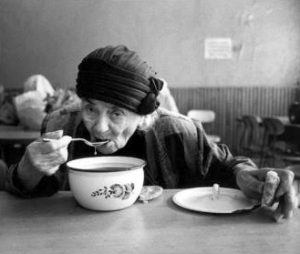The image is a grainy, aged black-and-white photograph capturing an elderly, frail-looking woman, likely in her 80s, sipping soup from a large ceramic bowl at a table. She wears a black hat adorned with a bow and a loose, raggedy jacket over a plaid shirt. Her left hand holds a biscuit or piece of bread, complementing the soup. The bowl has a matching white lid with a handle, placed on the table to her right. Her hollowed cheeks and thin frame emphasize her age. Behind her, a gray wall with wainscoting at the bottom and a small, unreadable white sign adorns the background. The room contains additional tables and chairs with round backs and metal legs, one of which has bags on it. Another person can be seen in the background, sitting at their own table.